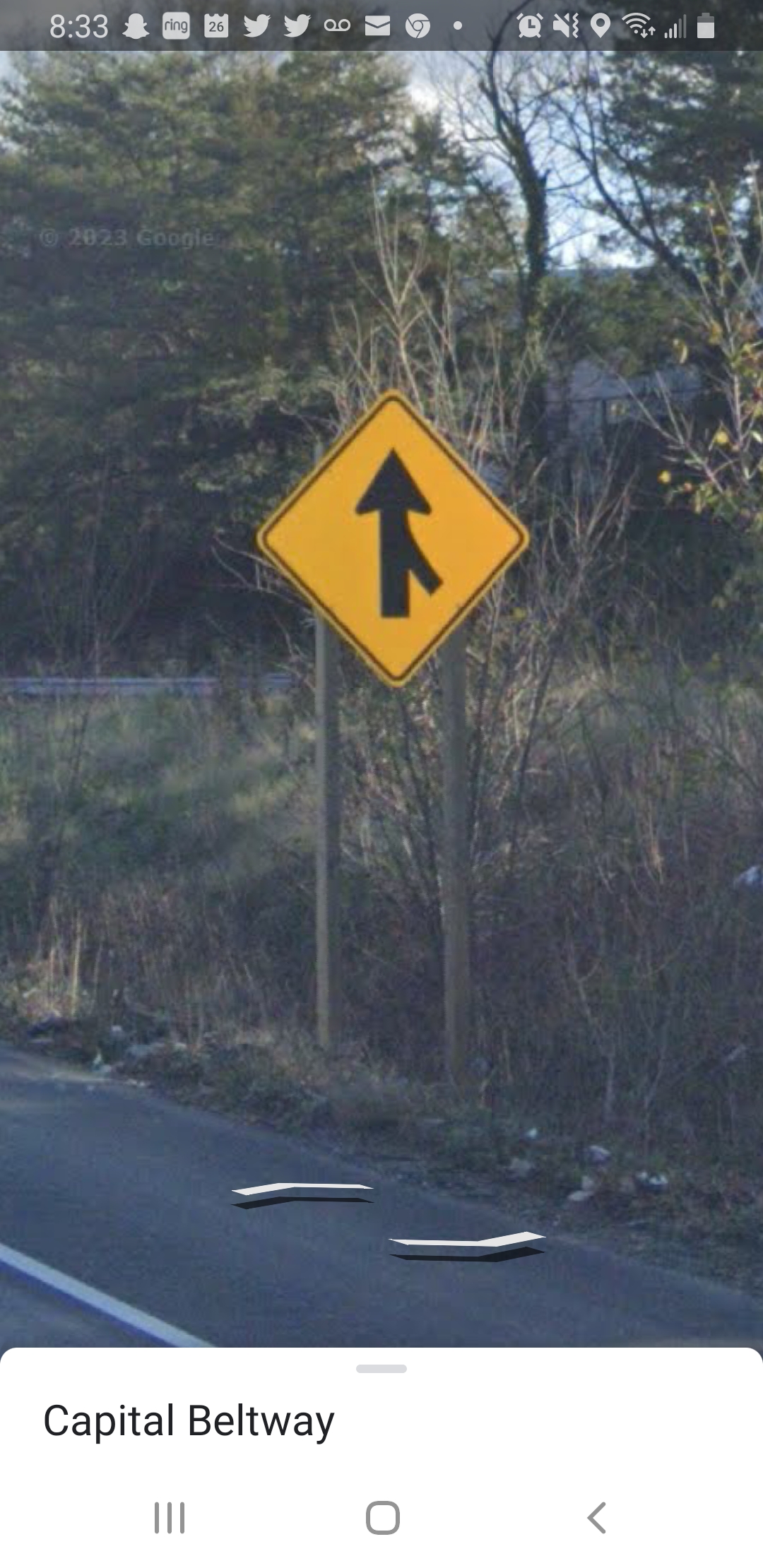The image captures an outdoor scene alongside a roadway, prominently featuring a diamond-shaped yellow road sign. The sign, bordered with a single black line, displays a black arrow pointing upward with an additional line merging from the right side, indicating a merging lane. Interestingly, the road sign appears to be floating, as no signpost is visible. Below, the dark asphalt road showcases two white arrows, also seemingly suspended, as shadows can be seen beneath them. The foreground and background are lined with lush green trees, contributing to the scenic atmosphere. The sky above is clear with a hint of blue, rendering the scene bright and airy. Below the image, text reads "Capital Beltway." Additionally, the snapshot seems to be taken from a phone, suggested by the visible status bar at the top, displaying various icons such as time, battery, and signal strength.